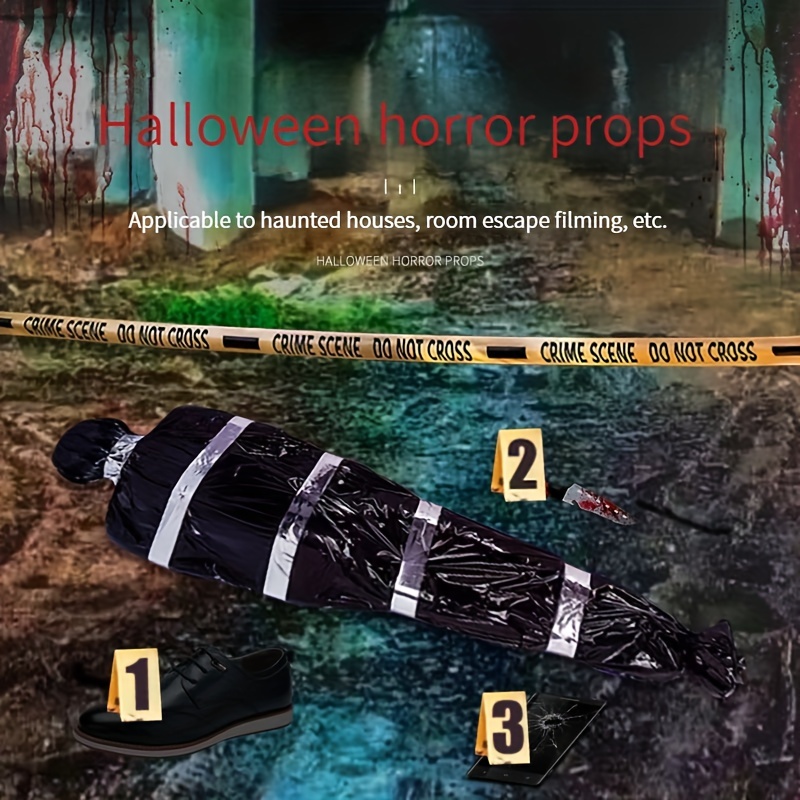This advertisement for Halloween horror props features an unsettling scene depicted to create a chilling ambiance. At the top, in bold red letters, it reads "Halloween Horror Props." Just below, in white text, it states "applicable to haunted houses, room escape filming, etc." The background resembles the interior of an abandoned building with eerie, dark greenish walls streaked with blood stains. Dominating the center of the image is a grim setup: a tunnel leading to a crime scene cordoned off with bright yellow "do not cross" police tape. On the floor lies a body wrapped in black plastic secured with silver duct tape. Surrounding the body are evidence markers labeled 1 to 3. Marker 1 is placed next to a black shoe, marker 2 is beside a bloody knife, and marker 3 is near a smartphone with a bullet hole through it. The haunting visuals are effectively designed to convey horror and suspense, making it ideal for any Halloween-themed event or attraction.